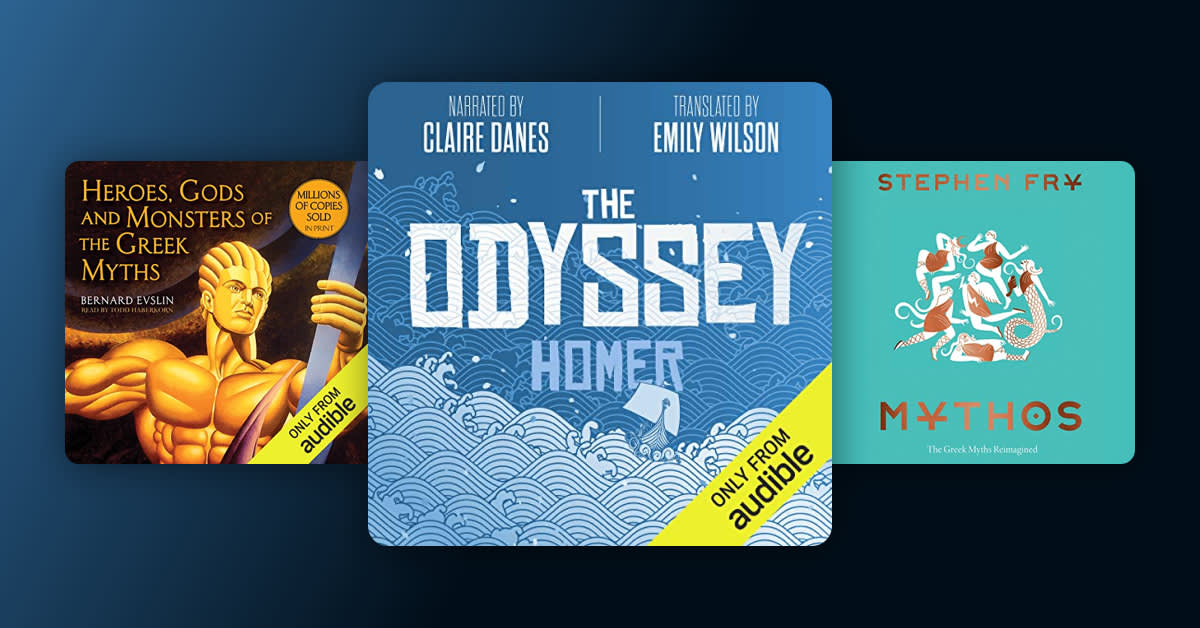This image portrays three distinct Audible audiobook covers set against a bicolored background, transitioning from solid blue on the left to black on the right. In the foreground, a prominent square cover showcases "The Odyssey" by Homer, framed with white text on a blue background featuring geometric wave designs and a Greek-style ship. This edition, narrated by Claire Danes and translated by Emily Wilson, includes a diagonal yellow banner in the bottom right corner saying "Only from Audible."

On the left, a smaller cover titled "Heroes, Gods, and Monsters of the Greek Myths" by Bernard Evslin depicts a muscular gold Greek statue grasping a purple rod. This cover has a yellow seal claiming "Millions of Copies Sold in Print" and another "Only from Audible" banner.

On the right, the third cover titled "MYTHOS" by Stephen Fry in gold text rests against a green background. The title's typography is distinctive, with the 'Y' shaped like a yen symbol and the 'O' resembling a target. The subtitle "The Greek Myths Reimagined" appears in white, beneath an array of six Greek mythological characters, including a mermaid and a winged cherub. Together, these audiobook covers represent a curated selection of Greek mythology-themed narratives available exclusively from Audible.